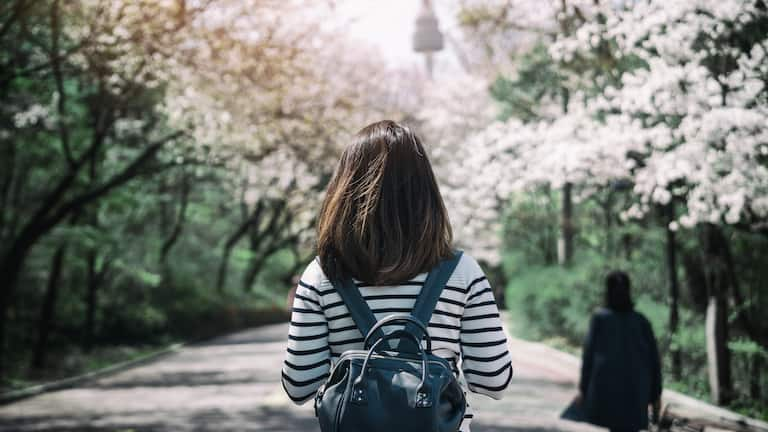This high-quality color photograph features a scenic walkway lined with blooming white dogwood or cherry blossom trees arching towards the top. The focal point is a woman with shoulder-length dark brown hair, walking away from the camera on a stone pathway. She is wearing a white shirt with black or blue stripes and carries a blue or black leather backpack. Another individual, dressed in dark clothing with dark hair, walks slightly ahead and to the right, appearing blurred. There are no other people visible on the path, and the serene setting emphasizes the peaceful ambiance. The overall composition creates a sense of depth and tranquility.